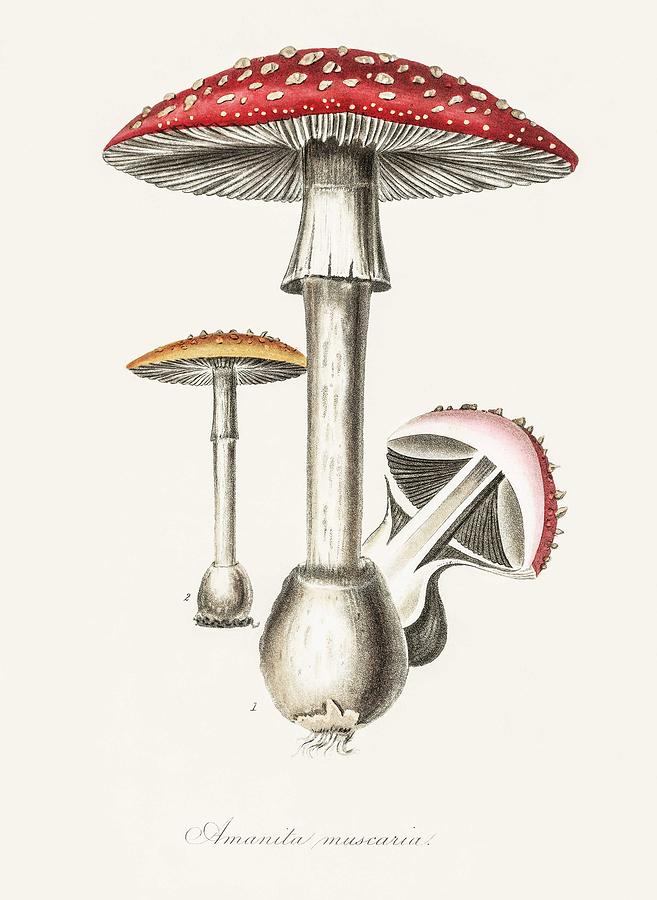This detailed image depicts an Amanita muscaria mushroom prominently displayed in the center, showcasing its distinctive large red cap adorned with white specks giving it a freckled appearance. The white, robust stem extends downward to an expanded, rounded base with visible root structures. Beneath the red cap, the gills are clearly visible, emphasizing its detailed anatomy. To the right, an earlier stage of the Amanita muscaria's development is illustrated. To the left of the prominent mushroom, an Amanita pantherina is illustrated, characterized by its yellow-orange cap with brown specks. The artwork is labeled with scientific names beneath each mushroom illustration, providing educational value. There is a faint shadow of a fallen red mushroom in the background, adding depth to the composition. The entire depiction is set against a slightly blurred, pinkish backdrop with a shadow of another red mushroom, enhancing the focus on the detailed mushrooms. An inscription in cursive, though a bit blurry, identifies the mushrooms and adds an artistic flair to the scientific illustration.